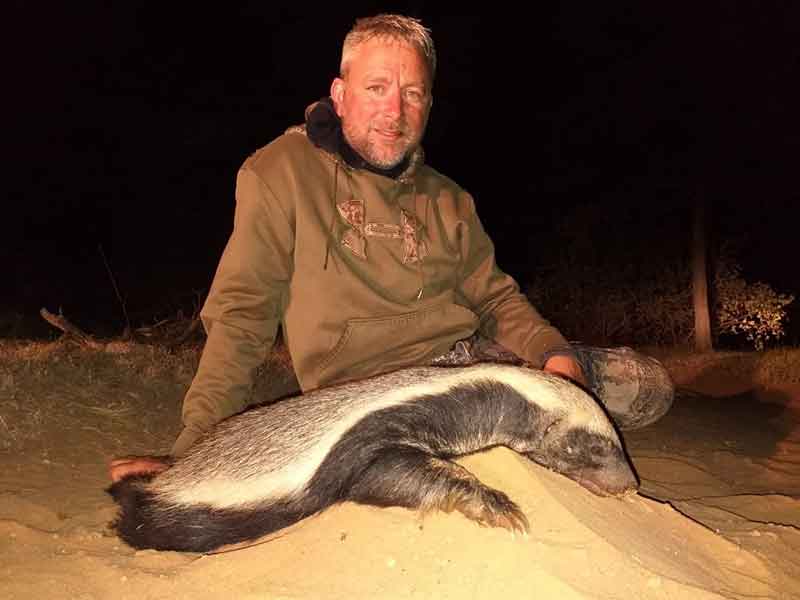In the image, a man with short blonde hair and a short stubble beard sits on the ground, looking directly at the camera. He wears a green hoodie with an "H" symbol on the front and two front pockets, along with camouflage cargo pants. His legs are bent at the knees, with his right hand resting on the ground and his left hand in his lap. The scene is illuminated by a camera flash, suggesting it's nighttime. 

In front of the man, on a small slope, lies a white-and-black honey badger, with white fur on its back and black fur around its sides. The badger has a short muzzle and one of its legs is visible sticking out on the ground. The setting appears to be a grassy area with a bush and trees to the man's right, contributing to the environment that resembles a nighttime safari or a setting in the African savanna.